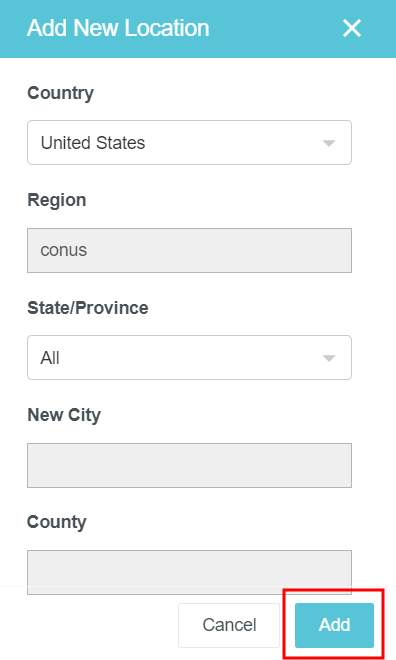The image appears to be a screenshot of a computer or cell phone interface, formatted vertically without a distinct border. At the top, there is a prominent blue bar with white text that reads "Add New Location." On the right side of this bar, a white 'X' icon is visible. Below this bar, there are several input fields designed for user interaction:

1. **Country:** A text field displaying "United States - State in the United States."
2. **Region:** A text field showing "CONUS."
3. **State/Province:** A text field with the content "All."
4. **New City:** An empty, gray text field.
5. **County:** Another empty, gray text field.

At the bottom right of the interface, there are two buttons:

- **Cancel:** A white button.
- **Add:** A blue button with white text that reads "Add." This button is outlined with a red rectangle.

The layout and color scheme suggest a structured and user-friendly form designed to input location details.